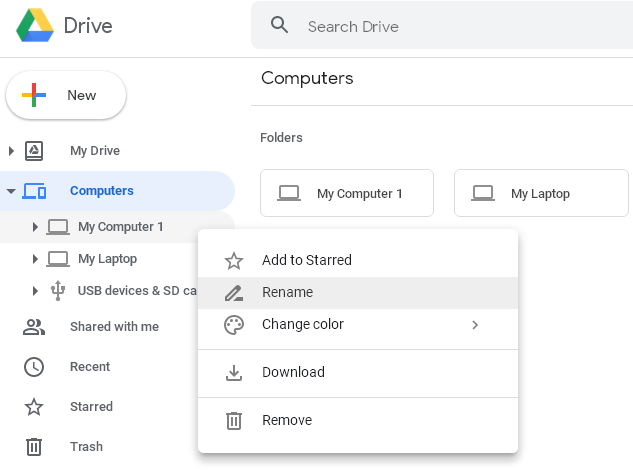This image is a cropped screenshot of the top left section of a Google Drive interface. The background is white, with the Google Drive logo prominently displayed at the top left corner. To the immediate right of the logo is a sizable search box labeled "Search Drive." Beneath this, a vertical panel on the left side categorizes various sections of Google Drive.

Highlighted in blue is the "Computers" section, indicating it is currently selected. The section's expandable subcategories are visible below it, with one of these subcategories actively clicked, likely under the "My Computers" group. This action prompts a pop-up box situated towards the bottom left of the screen. Within this pop-up, a list of five actions is displayed vertically. The second option, "Rename", is highlighted, guiding the user on how to rename subcategories within this interface.

This cropped screenshot serves as a visual guide for navigating the Google Drive interface to rename subcategories under the "My Computers" section.